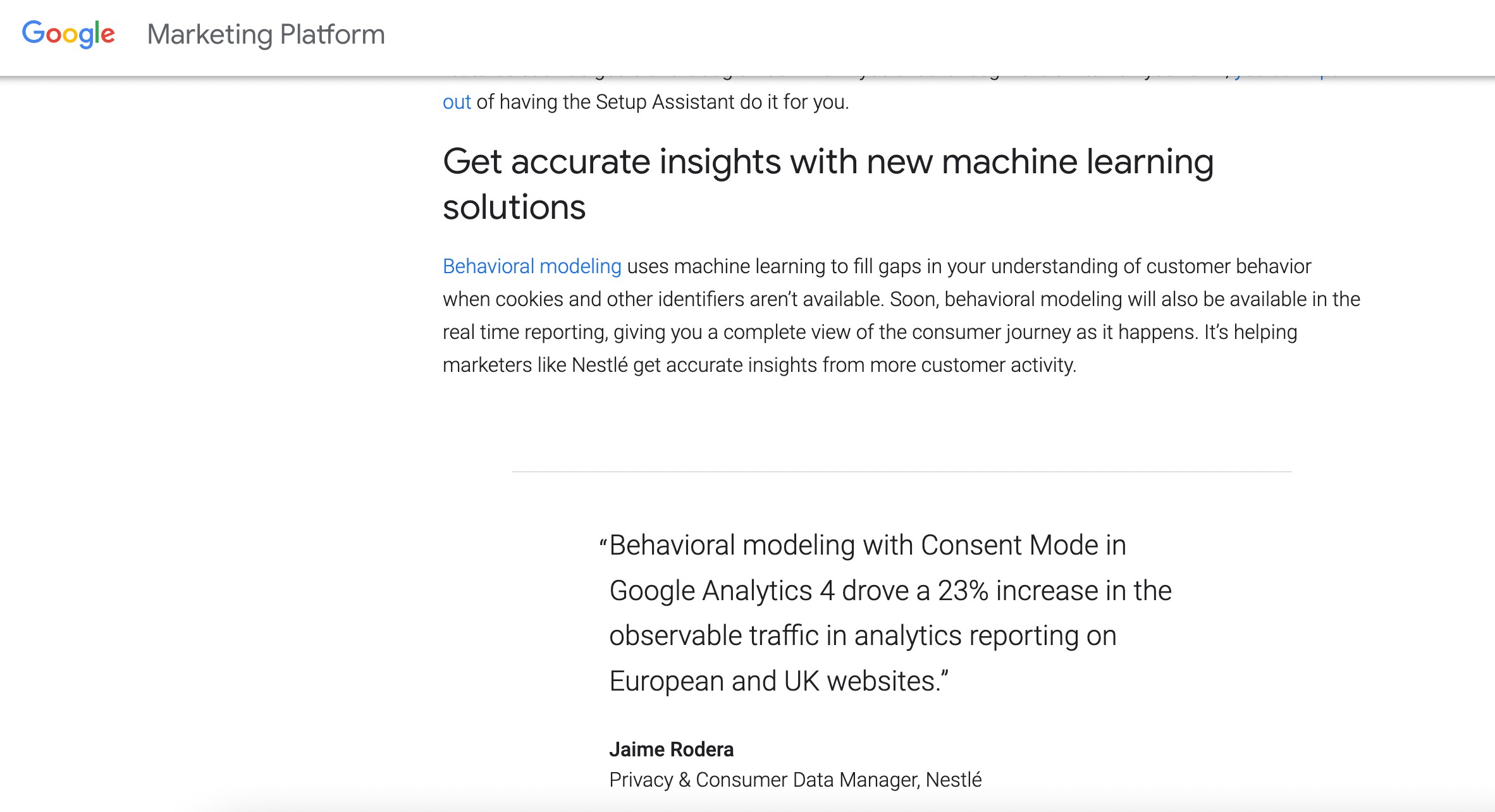The screenshot displays an informative interface of the Google Marketing Platform focusing on the integration of advanced machine learning techniques. 

Partially visible at the top is the headline, "Get accurate insights with new machine learning solutions," indicating the primary emphasis of the content. Just below this, a truncated phrase, "having the setup assistant do it for you," hints at automated assistance features.

The main body of the visible text elaborates on the concept of behavioral modeling. It explains that Google employs machine learning to bridge gaps in understanding consumer behavior when traditional data such as cookies are unavailable. Notably, it mentions that soon, behavioral modeling will extend to real-time reporting, thereby providing a comprehensive, immediate view of consumer interactions. 

An example provided highlights how this technology supports marketers. For instance, Nestle uses this machine learning capability to derive accurate insights from increased customer activity. The text continues, discussing the substantial benefits witnessed in behavioral modeling within Google Analytics 4, reporting a 23% increase in observable traffic on European and UK websites, attributed to this technology. 

A direct quote from Jamie Roddeera, Privacy and Consumer Data Manager at Nestle, underscores the practical and significant impact of these insights. 

Overall, the screenshot underscores the progressive strides taken by the Google Marketing Platform to enhance data accuracy and consumer understanding through sophisticated machine learning solutions.